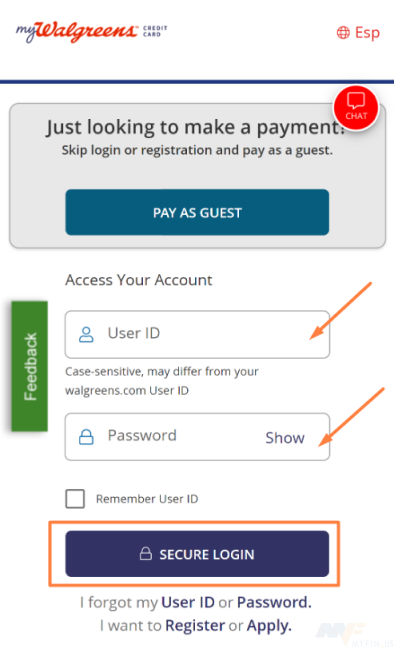The image is a screenshot of a Walgreens account registration page. In the top left corner, the text reads "My Walgreens Credit Card", and the top right corner features a globe icon with "ESP" next to it, indicating language options. Below this, there is a rectangular section with a grayish-blue background containing the message, "Just looking to make a payment? Skip login or registration and pay as a guest," followed by a blue "Pay as Guest" button.

A red circular icon with a speech bubble inside and the word "Chat" is overlaid on the image, indicating a chat support option. Below this, there is a header saying "Access your account" with a "Feedback" button next to it. 

The login section consists of a user ID text box with a red arrow pointing to it, highlighting the note: "Case-sensitive, may differ from your Walgreens.com user ID." Below this, there is another text box for the password, featuring a padlock icon and a "Show" option, with a red arrow pointing to it. 

An empty, unchecked square labeled "Remember user ID" is positioned beneath the text boxes. Following this is another rectangular button with a red border and a bluish-purple background. This button displays a white padlock icon and the words "Secure Login".

At the bottom of the page, the options "I forgot my user ID or password" and "I want to register or apply" are displayed.